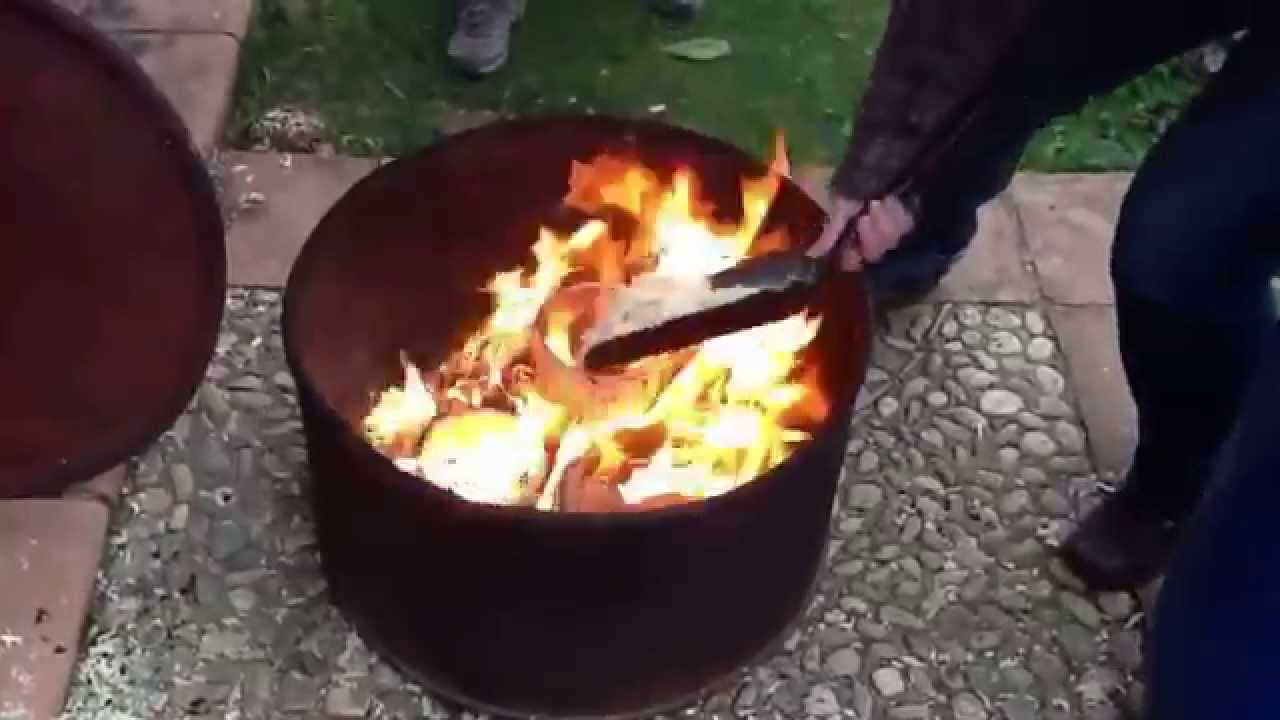This detailed, colored photograph, taken in landscape orientation, captures an outdoor scene featuring a large black metal vessel positioned on a stone walkway outlined with light-colored tiles. The vessel, resembling a massive bowl or cauldron, is filled with glowing coals and yellow flames. A matching lid lies off to the side. Surrounding the vessel are several indistinctly visible individuals; one person is bent over from the right, gripping a black tool resembling a tongue, while tending to the fire. Their knees and lower arm are visible, suggesting they might be stirring the coals or adding something to the container. You can also glimpse another individual’s foot in the upper left corner and a tennis shoe in the background, hinting at more people standing on the grass nearby. The entire scene is framed by the natural and meticulously detailed stone pathway, with a blend of representational realism.